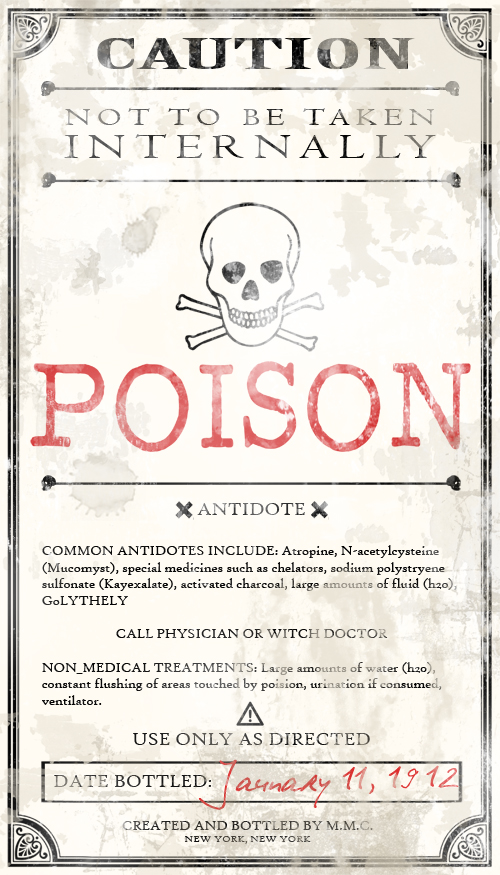The image is a black and white caution flyer with a black border and a rectangular, vertical layout. At the top, it prominently displays the word "CAUTION," followed by the warning "Not to be taken internally." Below this warning, there is a skull and crossbones symbol, under which the word "POISON" is written in striking red letters. Further down, in smaller text, flanked by X symbols on both sides, it says "Antidote." The flyer lists various common antidotes, although the specific names are difficult to decipher from the provided description. It advises to "Call a physician or witch doctor" for medical assistance, and includes non-medical treatments such as "large amounts of water" and "contact flushing of areas touched by poison." Continuing the instructions, it states "Use only as directed." At the bottom of the flyer, in red text, the date "January 11, 1912" is prominently displayed, and it notes that the content was created and bottled by "MMC, New York, New York." The entire piece has an old-fashioned appearance, suggesting it is a historical document related to poison safety.